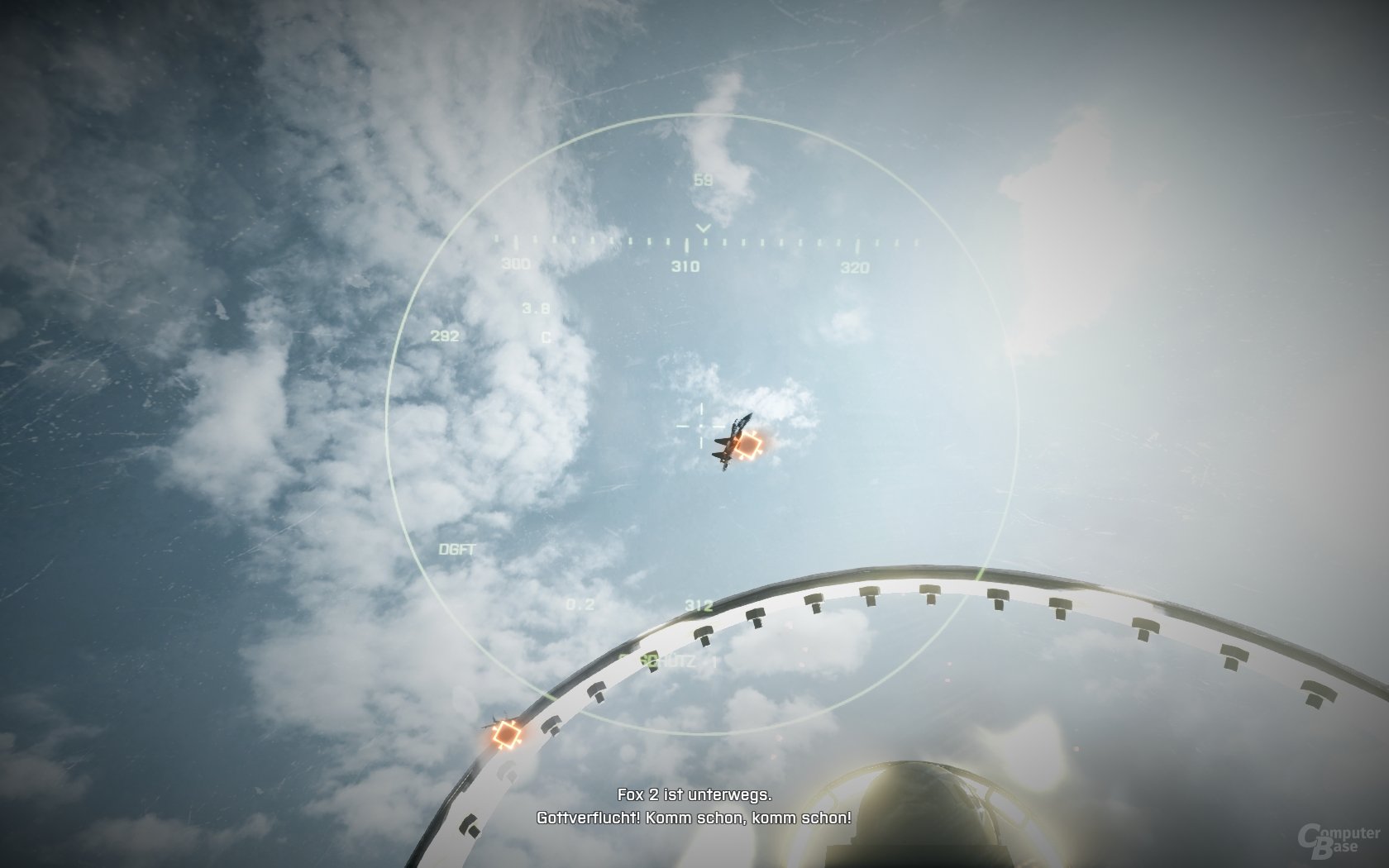The image features a light blue sky, subtly illuminated by sunlight emanating from the top right corner, casting a brighter shade of blue on the left side. At the bottom of the picture, a shiny golden sphere is radiantly lit, possibly reflecting the sunlight. This sphere is encased in a metallic arch. Moreover, a white bullseye surrounds a small black object in the sky, which could potentially be a plane, but its exact nature is unclear. An orange square marks this black figure, and another orange square is affixed to the metallic arch. Together, these elements create a visually intriguing composition.